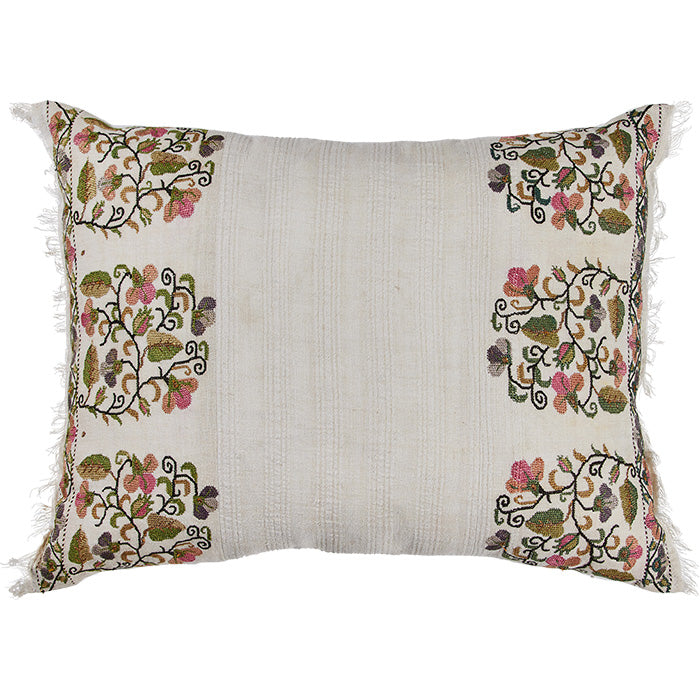The image shows a rectangular-shaped pillow with a somewhat weathered, off-white color, suggesting it may be older. The pillow is framed against a plain white background, which emphasizes its details. On both the right and left sides, there are patches of green and brown leaves interspersed with pink, purple, and orange flowers, forming a floral design that adds a touch of nature to the item. The fabric of the pillow is thick with a textured appearance due to vertical beige stripes in the center. Surrounding the floral patches and stripes are small, white tassels or threads hanging off the sides, enhancing its decorative appeal. The middle section of the pillow is blank, providing a contrast to the detailed edges. Overall, the combination of intricate floral patterns, textured stripes, and fringe detailing provides a rich visual interest to this seemingly timeworn pillow.